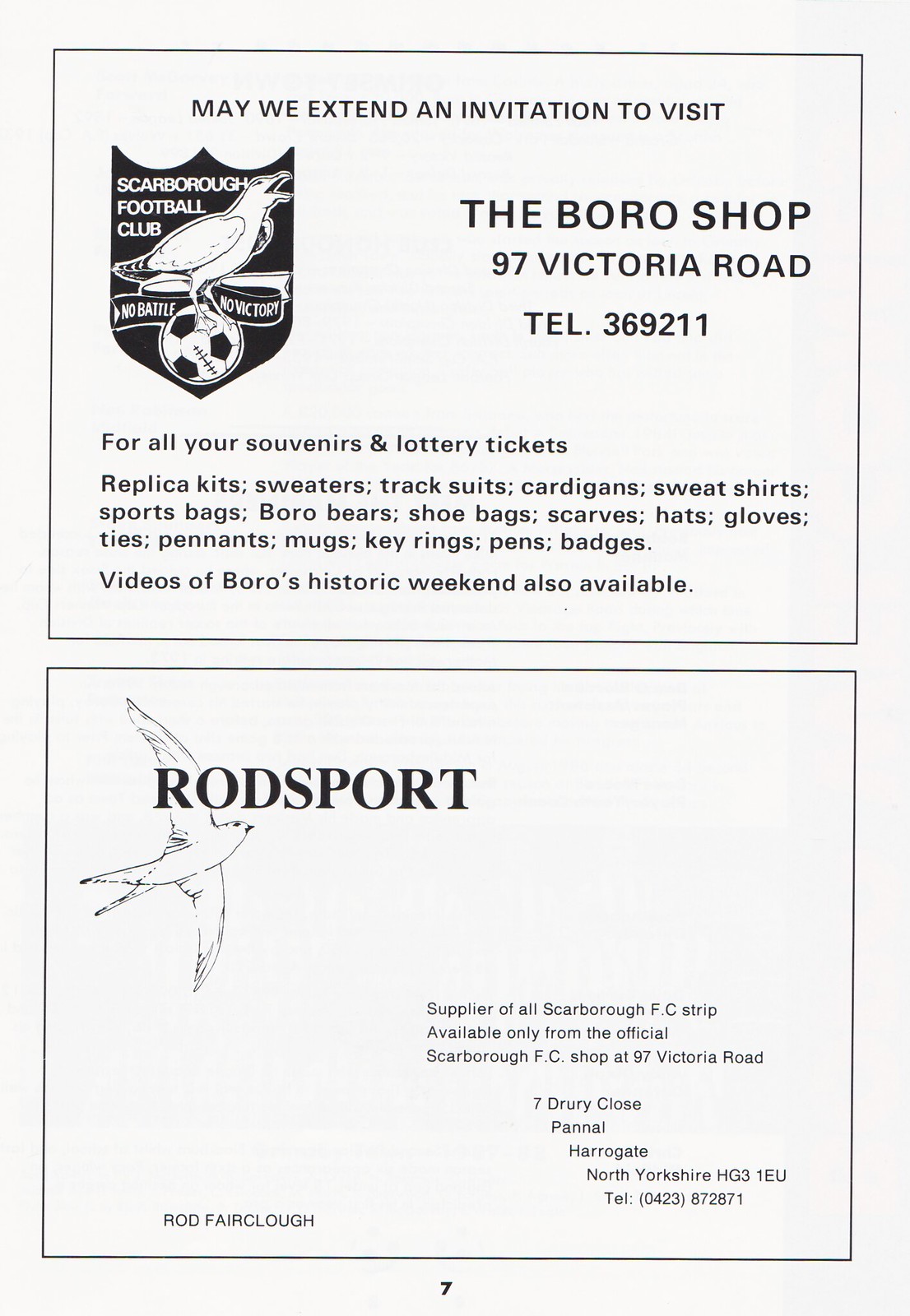In this black-and-white vintage magazine print, displayed on page 7, the image is oriented in portrait format and showcases two distinct, half-page advertisements enclosed in black frames. The top advertisement prominently features the Scarborough Football Club logo, depicting a bird perched on a soccer ball and the club's motto, "No Battle, No Victory." It extends an invitation to visit the Borough Shop at 97 Victory Road, providing a detailed list of available merchandise including souvenir and lottery tickets, replica kits, sweaters, track suits, cardigans, sweatshirts, sports bags, shoe bags, scarves, hats, gloves, ties, pennants, mugs, key rings, pens, badges, and videos of Borough's historic weekend.

The lower advertisement is for Rod Sport, which positions itself as the official supplier of all Scarborough FC team strips. This ad also includes a sketch of a bird and provides contact information for their locations at 97 Victoria Road and 7 Jury Clothes, Pannell, Harrogate, North Yorkshire, HG3 1AU. The overall layout and typography exude a classic, vintage print style reflective of the era.